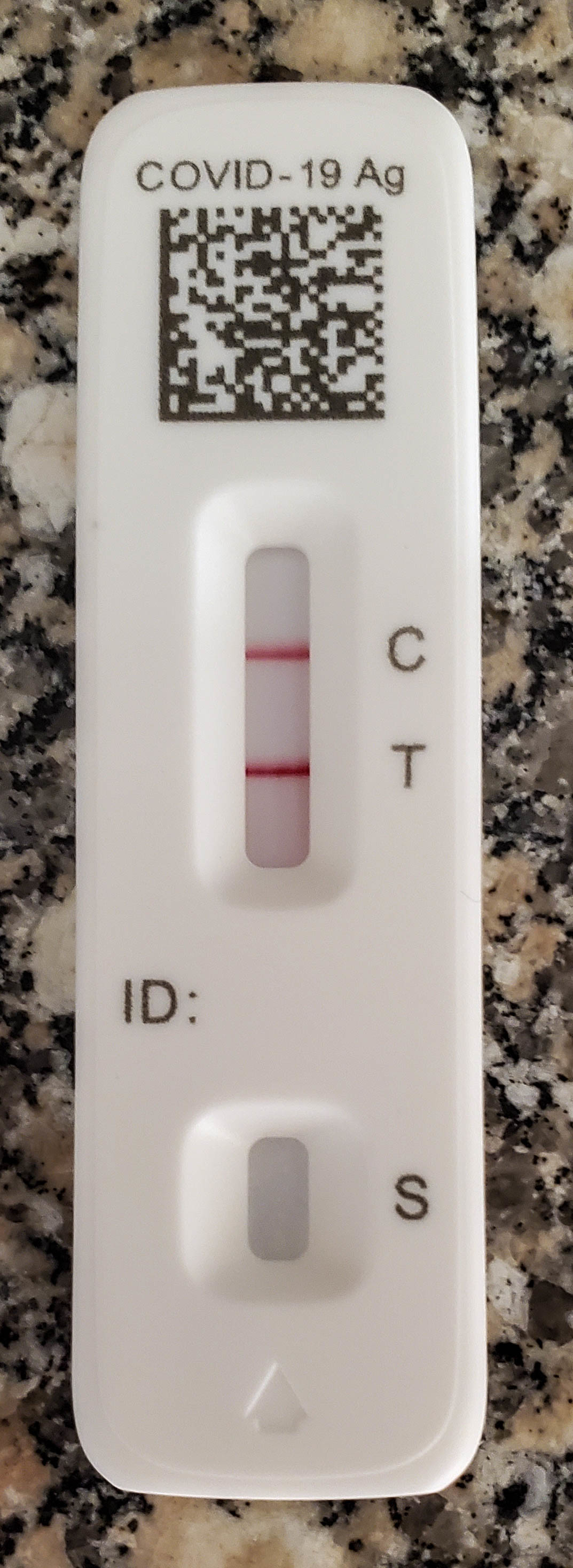This photo depicts a COVID-19 rapid antigen test kit prominently displayed on a dark granite countertop. The slim, white testing device is oriented vertically. At the top of the test, bold black letters read “COVID-19 AG.” Below, there is a recessed oval-shaped window featuring two distinct red lines. To the right, the upper line is labeled with a "C" (control line) and the lower line with a "T" (test line), both marked in black letters. Further down, an area labeled "ID:" appears empty, set within a smaller inset space, approximately half the size of the first window. Adjacent to this section, there is a letter "S" next to an indented arrow pointing upward towards the test windows. The countertop backdrop consists of an intricate mix of black, beige, and white hues, with black being the most prevalent color, emphasizing the sleek design of the test against the polished stone surface.